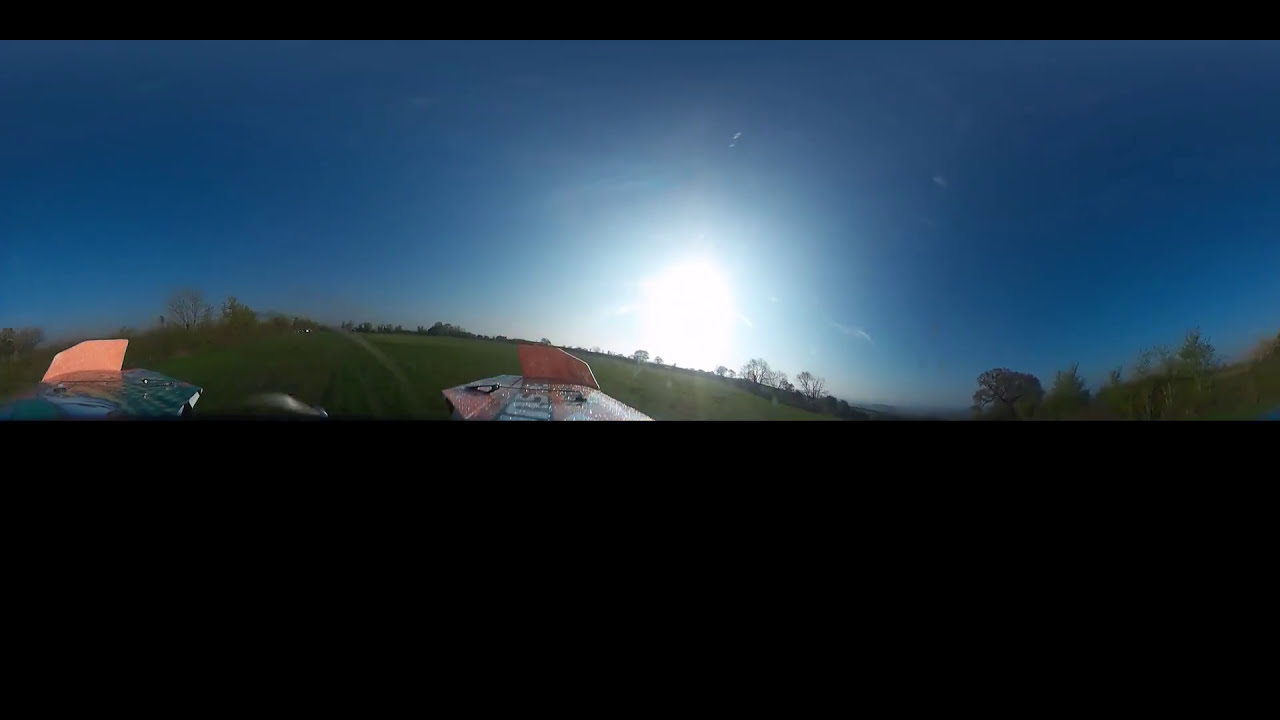In this image of an evening landscape, the bottom half is completely blacked out, creating a striking contrast with the richly detailed upper half. The scene features two green hills: a large one on the left and a smaller one on the right, with a road running between them. At the top of these hills, small trees dot the horizon. Dominating the foreground are two mysterious, wing-shaped objects that appear to be parts of an aircraft—a horizontal wing and a vertical orange fin with some indistinguishable lettering, possibly indicating the tail of a plane. The orange fin has a sparkly quality, adding an unusual detail. The sky above is a deepening dark blue, gradually darkening as evening sets in, with the sun glowing just above the horizon, casting a serene light over the landscape. The sky is mostly clear, with only slight traces of clouds, amplifying the overall tranquility of the scene.